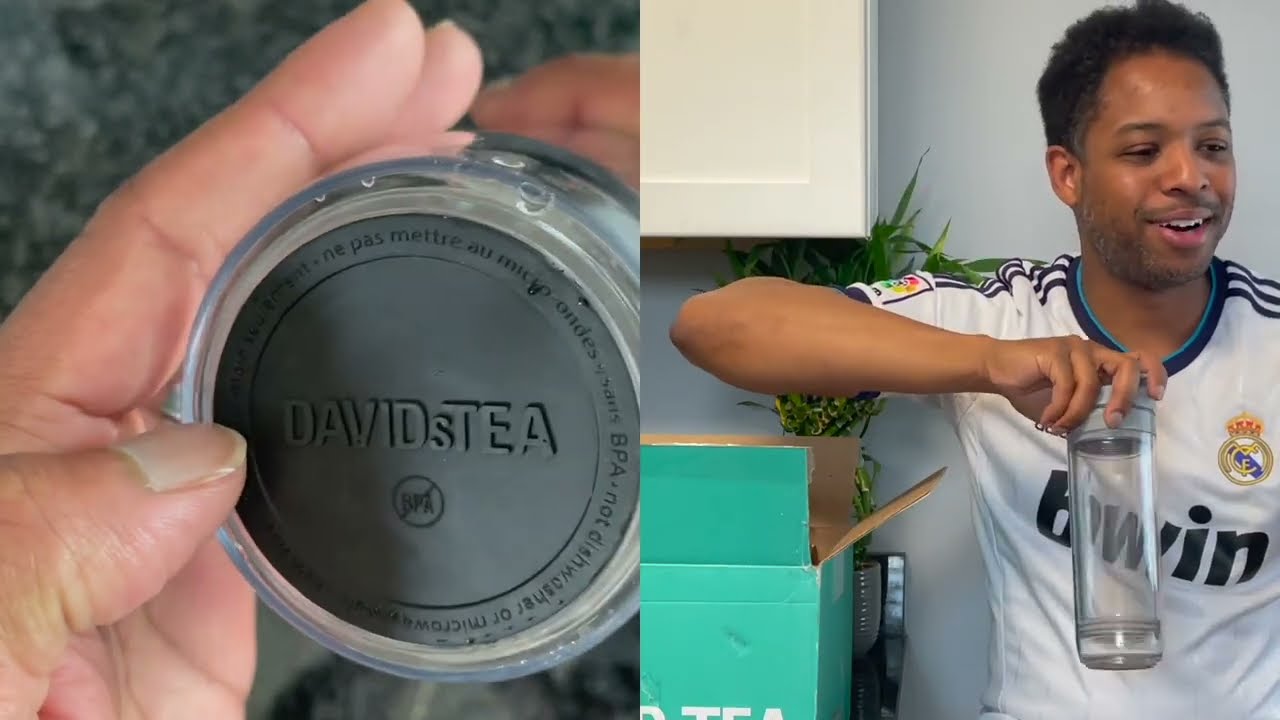The image is a composite of two pictures placed side-by-side. On the right side, a man with brown skin and short, graying black hair, is wearing a white soccer jersey with blue stripes on the shoulders. His jersey has the word "BWIN" written in black letters. The man is holding a clear container, possibly filled with water, which he seems to have just taken out of a teal or seafoam green box next to him. The background features a light gray wall with a white cabinet and a green plant. 

On the left side of the composite, an up-close shot shows a Caucasian person's hand holding a circular object with a black base. The writing on the base reads "David's T" in large capital letters, with a smaller "s". Beneath this, there is a symbol indicating "BPA-free" inside a circle with a cross through it.